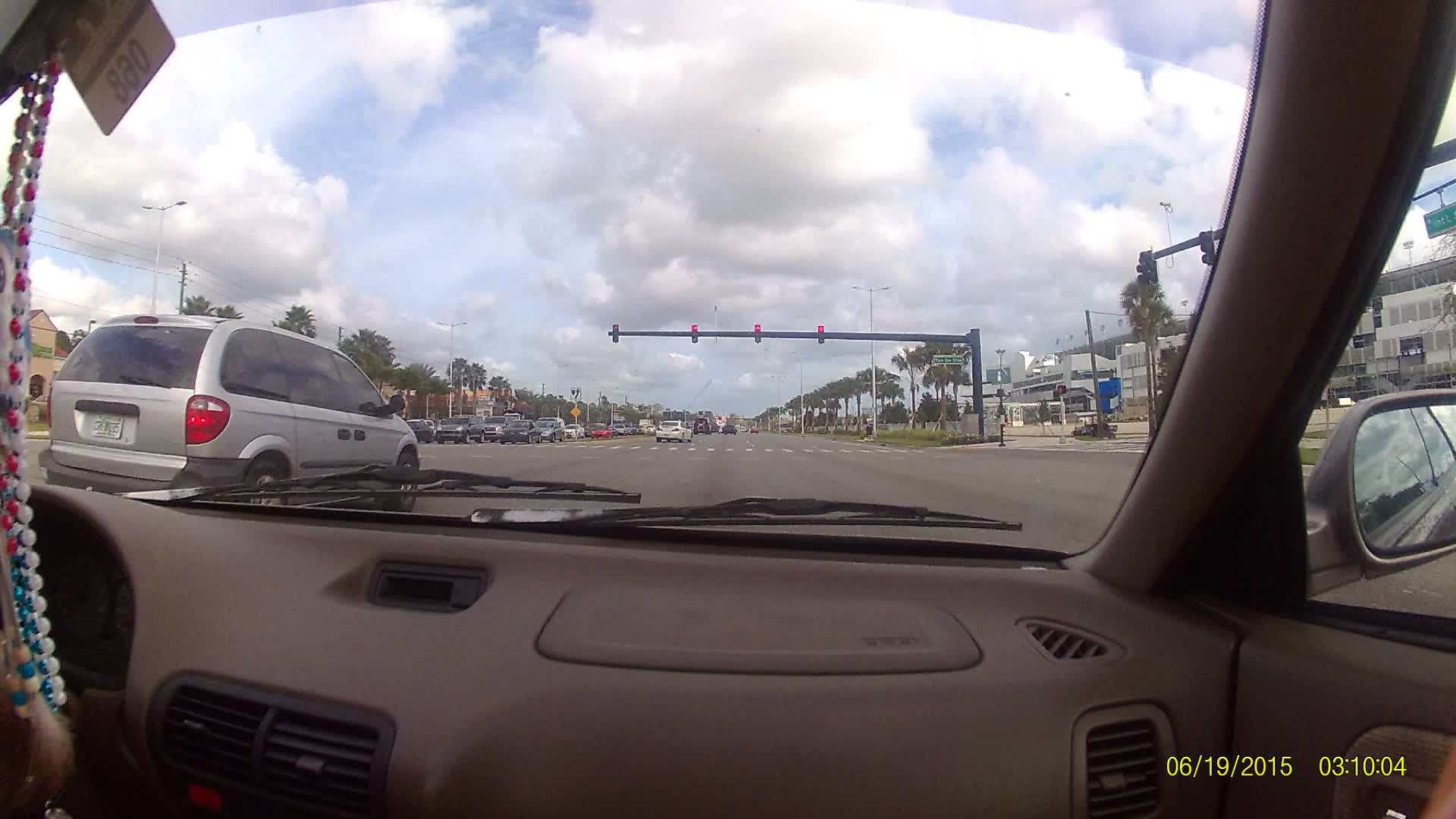The photograph, taken from the front passenger seat of a car with a gray interior, captures a detailed view through the windshield and side passenger window. The rearview mirror prominently features hanging beads in red, blue, and white, as well as a hang tag numbered 068. The car’s dashboard, including air vents and a hint of the black steering wheel, is visible. An overlaid yellow timestamp in the lower right corner shows the date 06 19 2015 and time 03 10 04. 

Outside, a wide road stretches ahead with a red stoplight and crosswalk dominating the view. A silver minivan is situated slightly ahead to the left. The sky is a vibrant blue interspersed with heavy, fluffy white and gray clouds. Street signs and buildings are seen on both sides of the road, with tall trees, potentially palm trees, lining the street and adding a touch of greenery to the urban landscape. To the right, a paved area and some grass are discernible in the distance, hinting at a car parking region amidst minimal traffic.